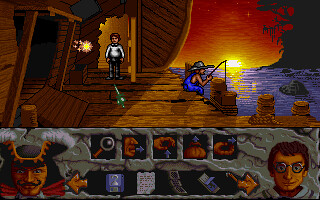The image depicts a cartoon-style screenshot from a video game, set against a scenic backdrop of a dock at either sunrise or sunset—characterized by striking amber and blue hues. The dock, constructed of wooden planks and pylons, features a wooden building or ship moored beside it. At the top of the image, a person wearing a white shirt, blue pants, and sporting brown hair stands in an illuminated doorway, with a silver sword visible in front of them and a star-like sparkle nearby. To the right, another individual, dressed in blue overalls and a significant hat, sits on the edge of the dock, engaged in fishing as their line dips into the water. The foreground of the image includes a gameplay interface: the bottom left corner shows a pirate captain with shoulder-length black hair, a black and gold hat, and a thin mustache, while the bottom right displays a pale-skinned man with brown hair and glasses. Between them are several boxes depicting various tools—a spyglass, a person's mouth with an arrow, and a hand with an upward arrow—accompanied by additional tools beneath, with arrows for scrolling through more items.